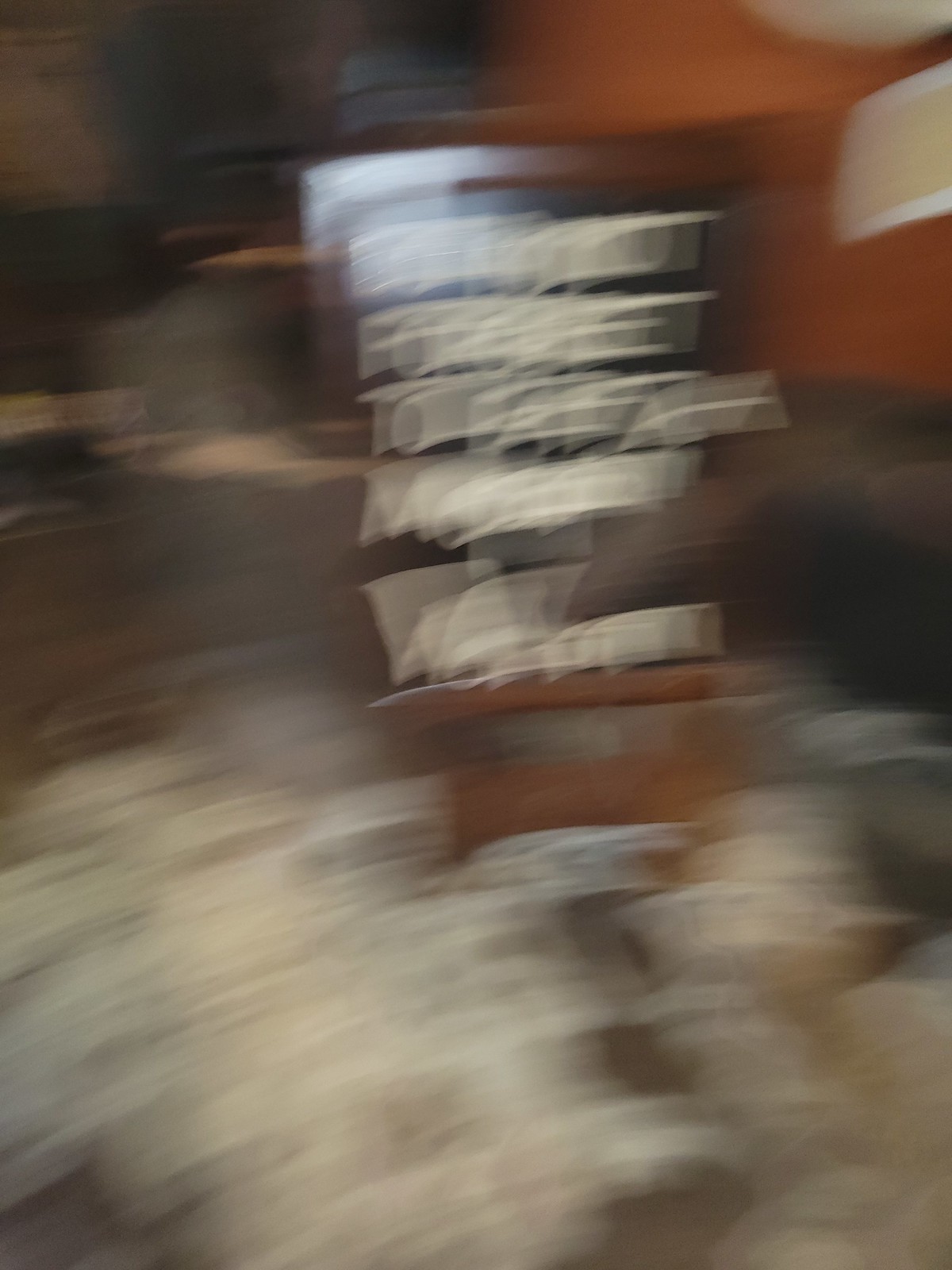A severely blurred photograph showcasing an indiscernible sign, seemingly captured mid-shake, resulting in extreme motion blurring. The sign features an off-white font against a black background, surrounded by orangey red-brown wood. The ground level depicts indistinct white shapes, some with striped patterns and floral-like designs. An orange wall is partially visible in the background, along with a black structure behind the blurry sign. The overall image is heavily distorted, making it difficult to discern specific details.